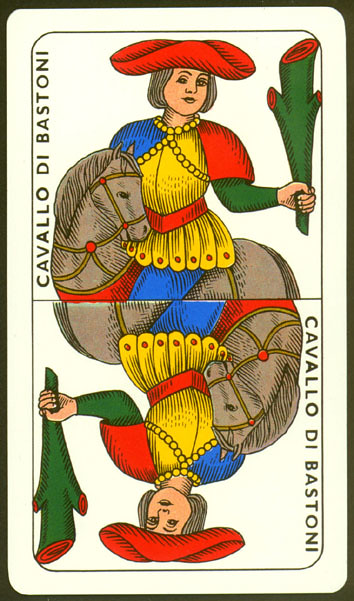This image appears to be a detailed depiction of a card, possibly similar to a playing card or tarot card. The background is stark white, framed by a black border with an additional fine line just inside, creating an inner box with curved edges. The card features symmetrical designs on the top-left and bottom-right, both sections displaying the text "Cavallo di Bastoni," which translates to "Knight of Clubs" in some card decks.

At the center of the card is a man seated on a horse. The man has distinct features including a gray-haired head beneath a bold red sombrero-like hat. His attire is primarily gold but includes distinct colored elements: a blue left shoulder, a red right shoulder, a red belt, and red jeweled accents along the skirt of his outfit. He dons blue pants, which add another layer of contrast to his vibrant clothing.

The horse he rides shares a similar aged elegance with gray hair and is adorned in gold-reined tack embellished with red jewels identical to the man's outfit. The horse itself is draped in a red garment, matching the thematic color scheme of the card.

The man holds a peculiar green object, resembling a cactus with red swirling patterns, as if the ends and arms were sliced open to show a detailed inner structure. This intricate design element adds an air of mystery and complexity to the card, aligning with the traditions of illustrative, symbolic card designs.